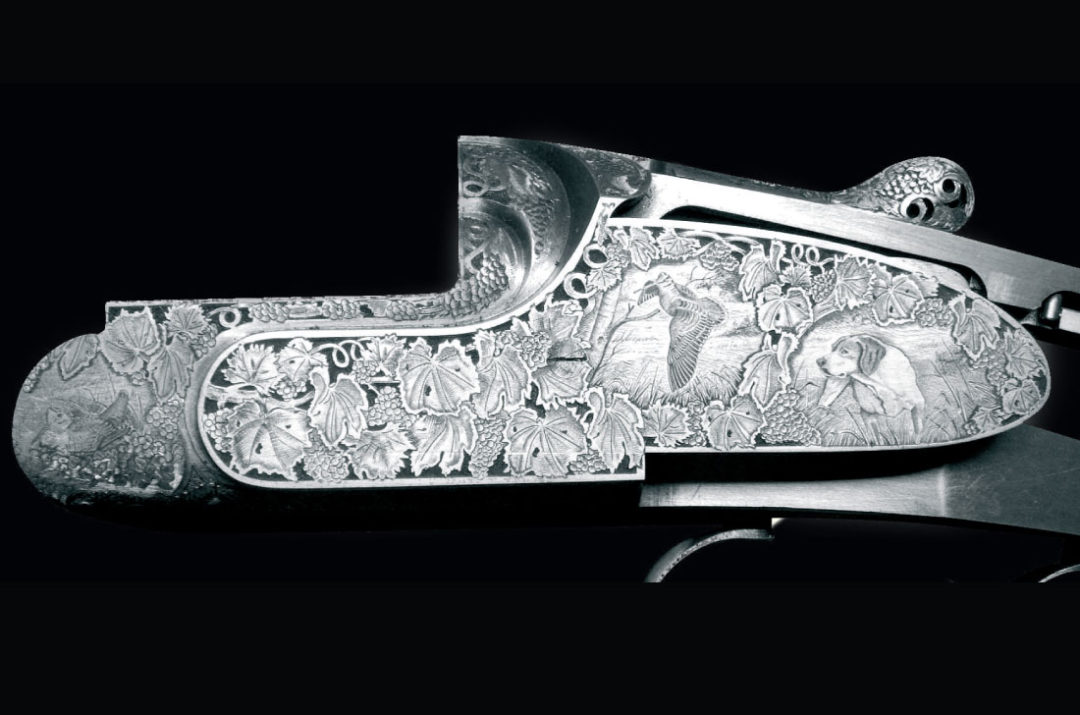The photograph features a silver, irregularly-shaped metallic object that somewhat resembles the shape of a shoe. It is set against a solid black background, which occupies most of the frame, highlighting the metallic sheen and intricate details of the object. The left side of the object is richly ornamented with carvings of leaves, featuring what appear to be images of a dog and a bird amid the leafy background. The top portion of the object includes a smooth, stainless steel lever that contrasts with the ornamental parts. This lever seems to make the object more flat and might be a separate component. To the bottom right, there is a smooth, slightly bent steel section attached to the ornamented area, adding to the irregular shape of the object. The emphasis on different textures and detailed carvings, set against the dark background, makes the object the focal point of the photograph, although its exact function remains unclear.